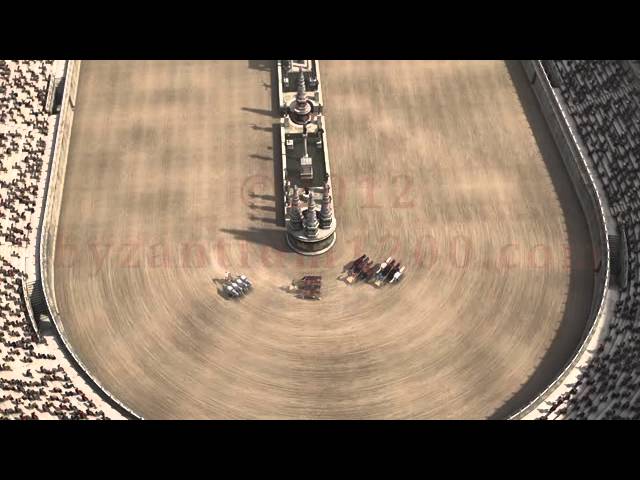An aerial photograph captures an intense chariot race on a large, oval-shaped horse racetrack, reminiscent of Roman era racing. Four chariots, each pulled by teams of four horses, can be seen navigating a sharp left turn on the track. The leading chariot, driven by black and white horses, is closely followed by a second chariot with black horses adorned with red saddles, and a third chariot also with red-saddled horses. Trailing behind, a fourth chariot is propelled by white horses. The expansive track features a central divider with towers, adding to the historical ambiance. The grandstands are filled with numerous spectators, engrossed in the race. A red, ink-styled watermark reading "Syzantium1200.com" and dated 2012 is faintly visible on the image, suggesting a historical reenactment or a scene from a period film.